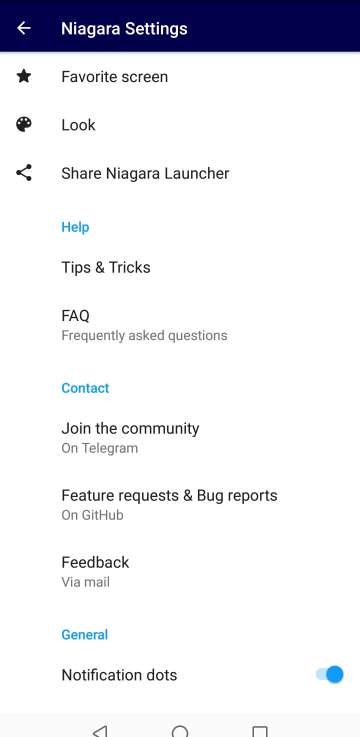Screenshot of the Niagara Launcher Settings Interface:

At the top of the mobile device screenshot, there is a prominent blue bar spanning the width of the screen. In the upper-left corner of this bar, a white arrow is visible. Centrally positioned on the blue bar is the title "Niagara settings."

The main section of the page beneath the blue bar features a white background. From top to bottom, a list of various settings is clearly displayed. The first setting, labeled "Favorite screen," is accompanied by a star icon on its left. Below it, the "Look" setting is marked by a paint palette icon, and the "Share Niagara launcher" option is identified with a share symbol.

Continuing down the page, there is a help section, which includes options such as "Tips and tricks" and "Frequently asked questions." Following this, a contact section provides multiple ways to connect, including "Join the community on Telegram," "Feature requests and bug reports on GitHub," and "Feedback via email."

The final section on the page is labeled "General." Within this section, the "Notification dots" feature is identified, which is currently turned on.